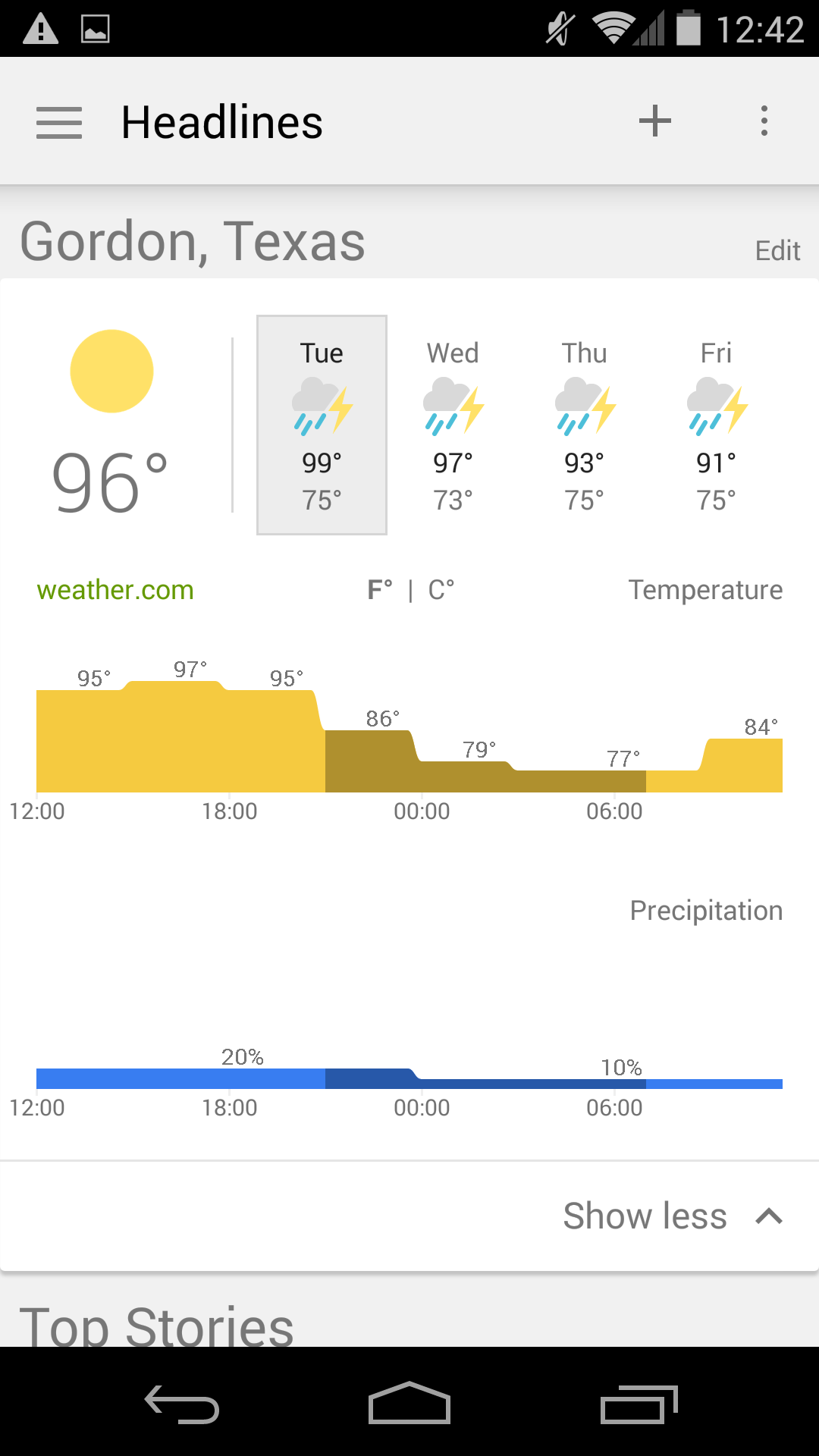This is a screenshot captured from a smartphone. At the top, there's a black bar displaying various small icons indicating the phone's network coverage, Wi-Fi signal, and the current time, 12:42. Directly below, on the left, is a hamburger icon, followed by the word "Headlines." A bit further down, the name "Gordon, Texas" is displayed, indicating the location. Underneath the location, the weather forecast for Tuesday, Wednesday, Thursday, and Friday is shown, with the current weather being sunny and 96 degrees Fahrenheit, as reported by weather.com.

Additionally, there's a detailed chart depicting the temperature changes from 12:00 PM to midnight and continuing into the next day. The chart also illustrates the expected rainfall and precipitation levels over this period, presented in bar chart format. Toward the bottom of the screenshot, a tab labeled "Show less" with an upward-pointing arrowhead is visible, likely intended to collapse the detailed weather information.